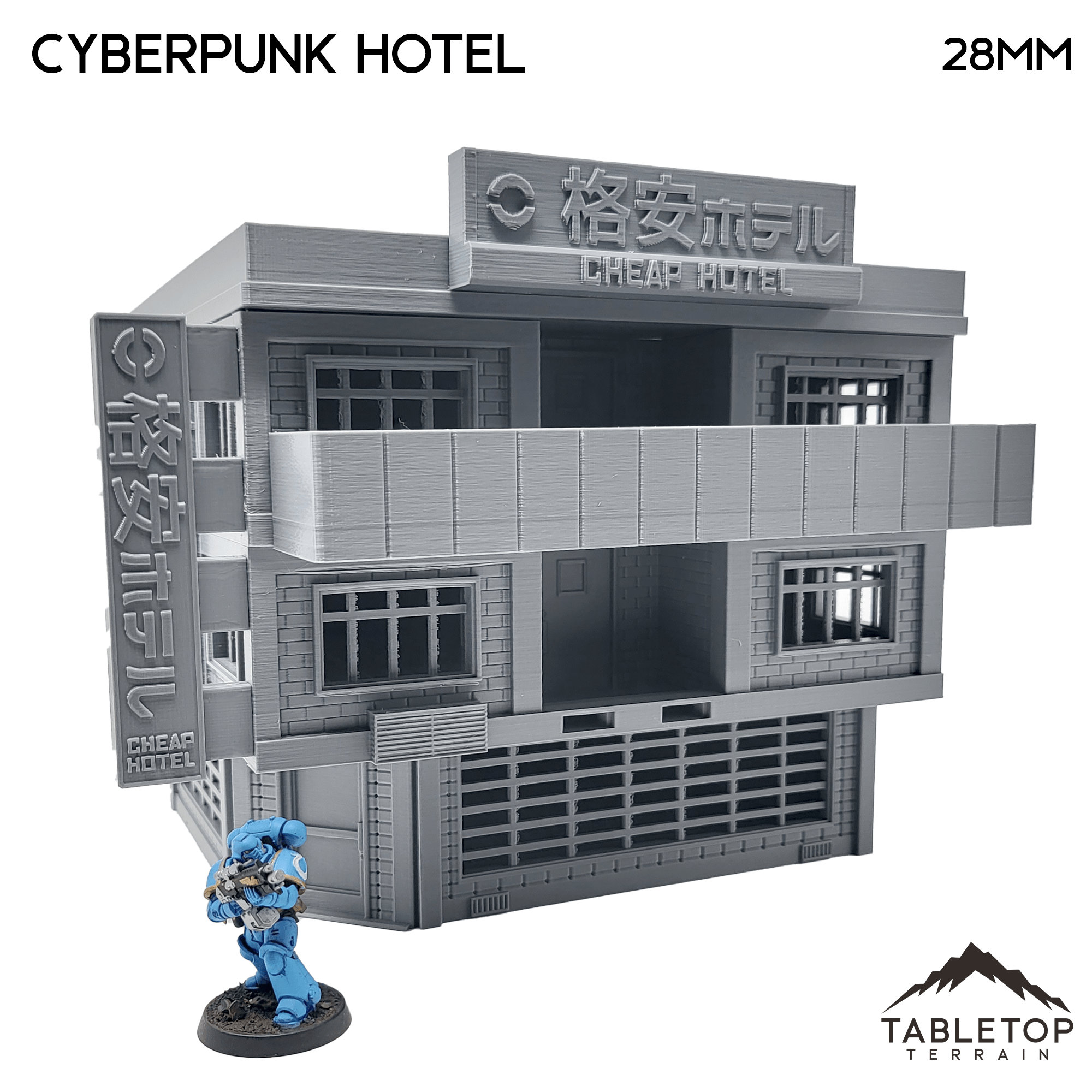The image depicts a detailed plastic model of a cyberpunk hotel, predominantly grey in color, and measuring 28 millimeters in length. The hotel, named "Cheap Hotel," is prominently marked with signs in both Chinese characters and English. It is a two-story structure featuring forward-facing windows—two per floor—with a balcony situated between the first and second floors. Below the main structure appears to be a parking garage. To the left of the building, there is a figurine dressed in a suit and holding a weapon, standing on a round block of plastic cement. Additionally, there is a blue tree, resembling a bonsai, situated in front of the hotel, on a grey base that matches the building’s color. In the bottom right-hand corner of the image, the "tabletop" logo is visible against a white background, suggesting the scene is part of an advertisement for a tabletop game.